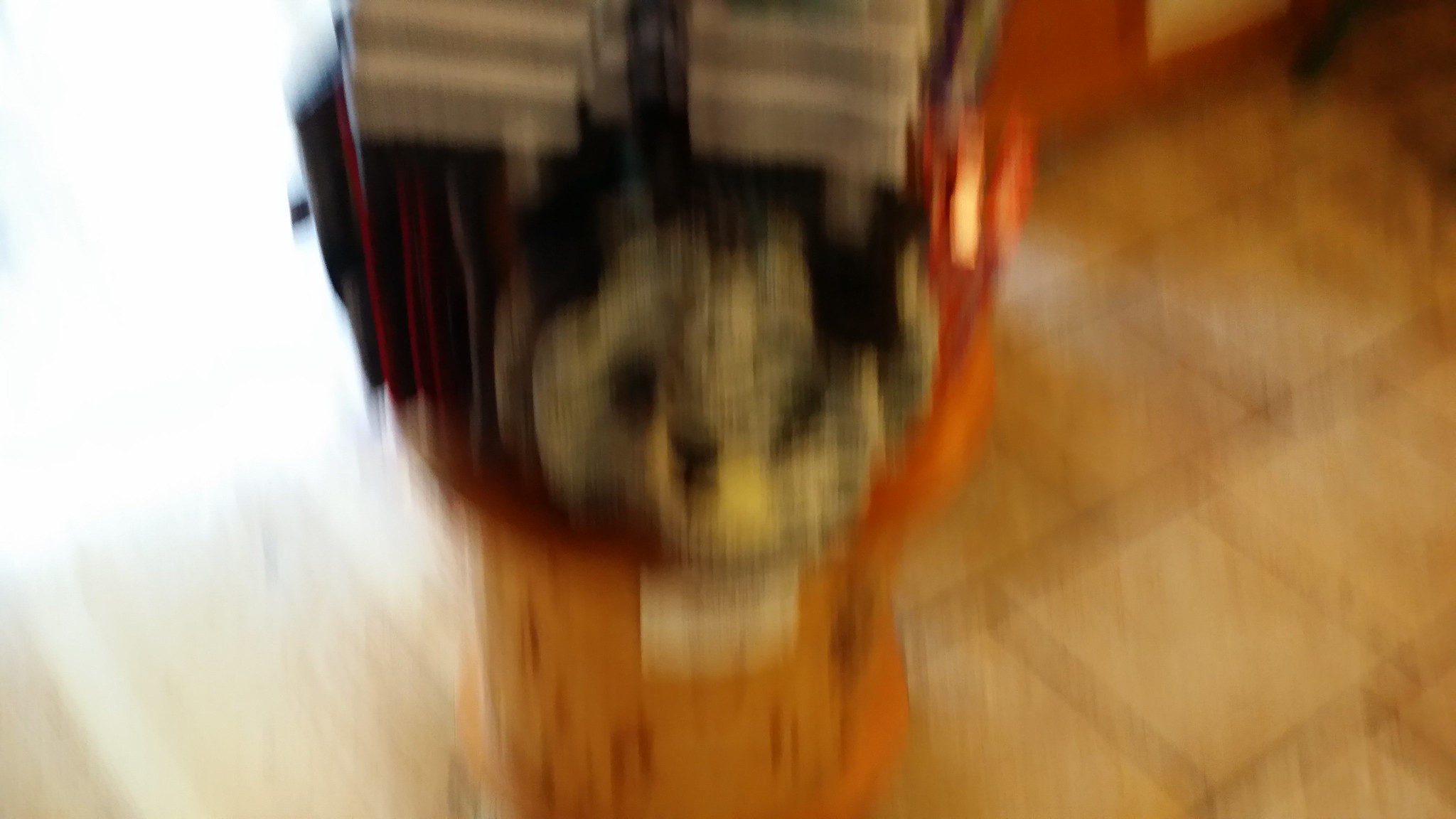A blurred, first-person perspective photograph captures a tiled room illuminated by a bright light source, likely sunlight, entering from the top left corner. In the foreground, positioned slightly above eye level, lies a cloth bucket containing various items of clothing. Notably, there is a yellow cylinder next to the bucket, possibly another container, revealing a red interior visible around its rim on the left side. Inside the bucket, there appears to be a beanie featuring a beer-themed design, along with pink and white striped scarves that extend out of the frame towards the top middle. The overall motion blurriness suggests the photographer took the image while in motion, adding a dynamic and somewhat chaotic element to the scene.